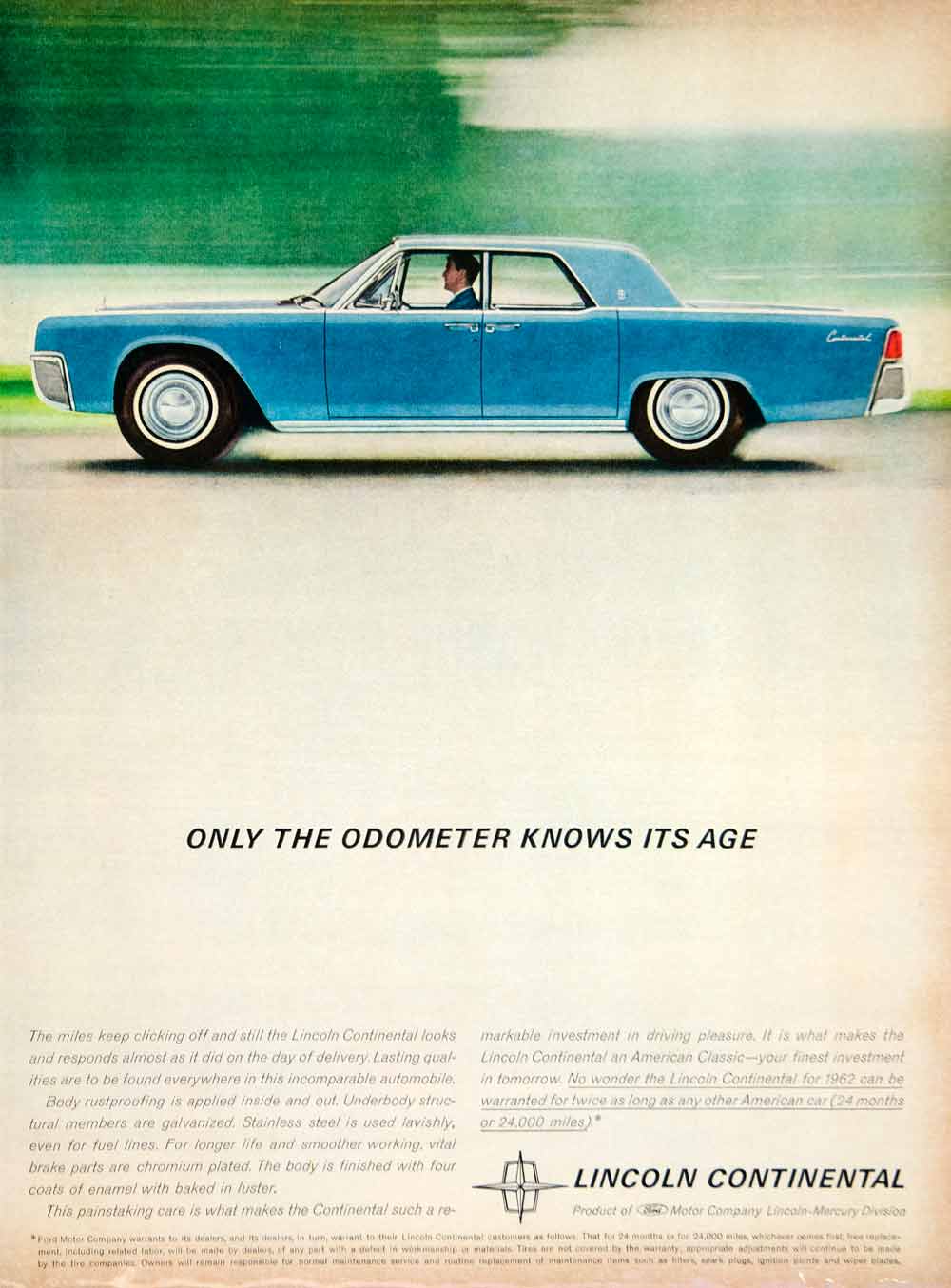The image depicts a vintage blue Lincoln Continental from the 1960s, specifically the 1962 model, being driven to the left by a man in a black suit. The car has a rectangular shape with a distinct top, likely a two-door model, featuring metal hubcaps with big silver centers and a small white ring around them. The background is a blend of blurred green trees on the left and a plain sky with distant trees on the right, giving the impression of speed. The top part of the image has a greenish background. Overlaying the image is the text "Only the odometer knows its age," emphasizing the car's enduring quality, along with faded gray text mentioning the lasting qualities of the Lincoln Continental. Below this text, "Lincoln Continental" is prominently displayed, hinting at an advertisement or promotional material for this classic automobile.